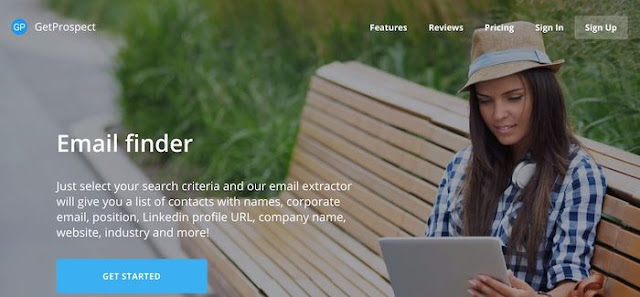**Front Page of Get Prospect Website**

The front page of the Get Prospect website features a visually engaging background image of a woman seated on a wooden bench beside a walkway. She is dressed in a blue and white checkered flannel shirt and a brown hat with a light gray strap around its crown. She is holding a laptop and intently looking at its screen. 

In the top left corner of the page, the Get Prospect branding is prominently displayed with the text "Get Prospect" beside a blue logo containing the white initials "GP." 

Along the left-hand side of the image, a brief description of the website's main service is provided in white text. It reads: "Email Finder. Just select your search criteria, and our email extractor will give you a list of contacts with names, corporate email, position, LinkedIn profile URL, company name, website, industry, and more." Below this description, there is a large blue "Get Started" button with white text.

In the upper right corner of the page, there are navigational options including a highlighted "Sign Up" button, alongside links for "Sign In," "Pricing," "Reviews," and "Features."